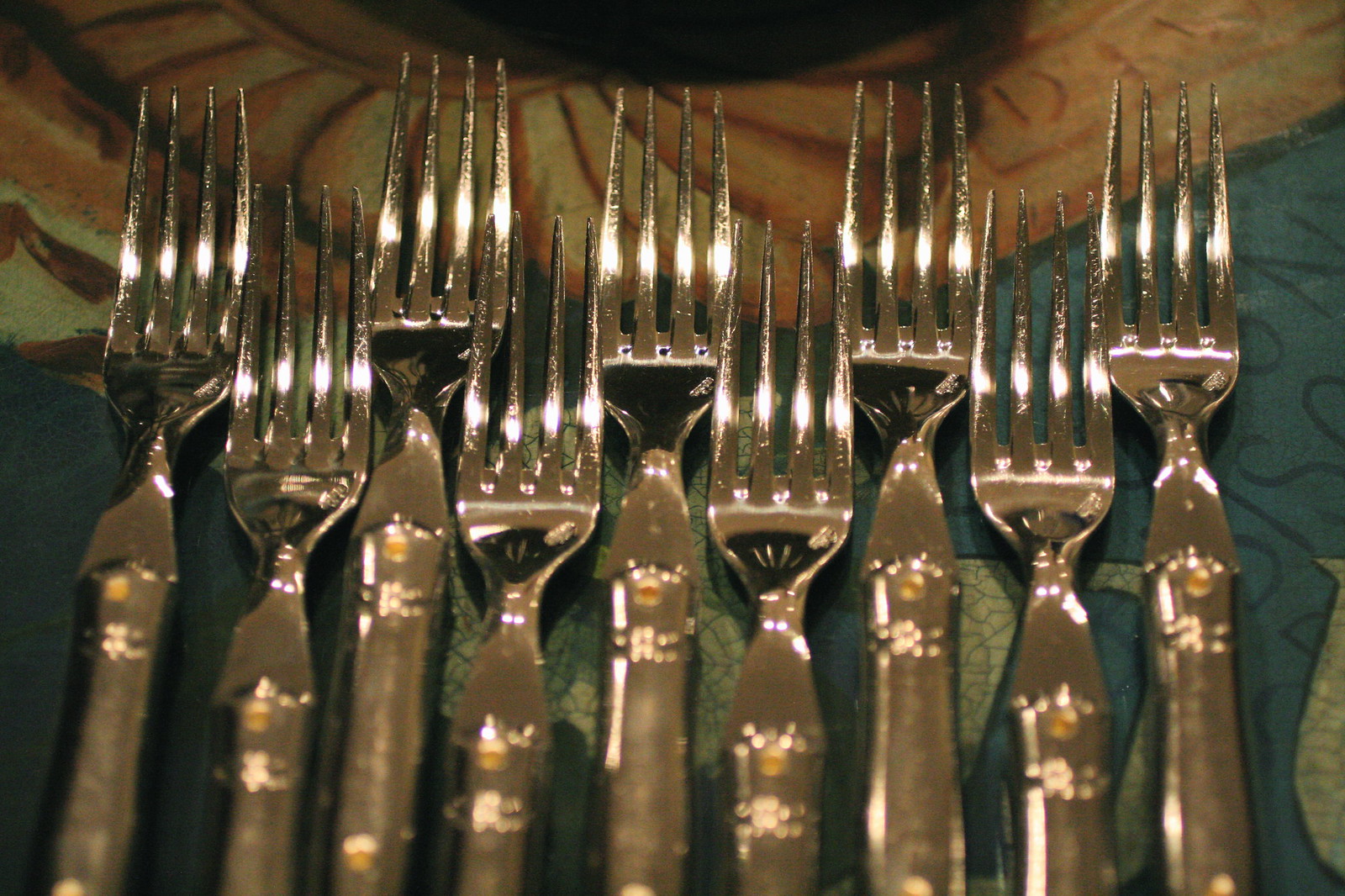This detailed, close-up color photograph captures nine exquisite, shiny silver forks meticulously arranged side by side on an ornate table setting. Each fork, elongated vertically with the tines facing up and the shafts extending downward, alternates in height—some extending nearly to the top of the image while others reach about 80% of that height. The intricate arrangement creates a rhythmic pattern of high and low, starting with a high fork on the left and ending with a high fork on the right.

The decorative etchings in gold at the top of each shaft hint at the forks' fine craftsmanship, despite being slightly blurred. The reflective surface of the forks captures glimmers of surrounding light, enhancing their elegance. 

The backdrop features a luxurious placemat or tablecloth displaying a blend of muted green, light brown, gold, and teal hues, enriched with intricate black and brown designs. This ornate setting suggests an ambiance of sophistication and timeless beauty, augmenting the refined appearance of the silverware.